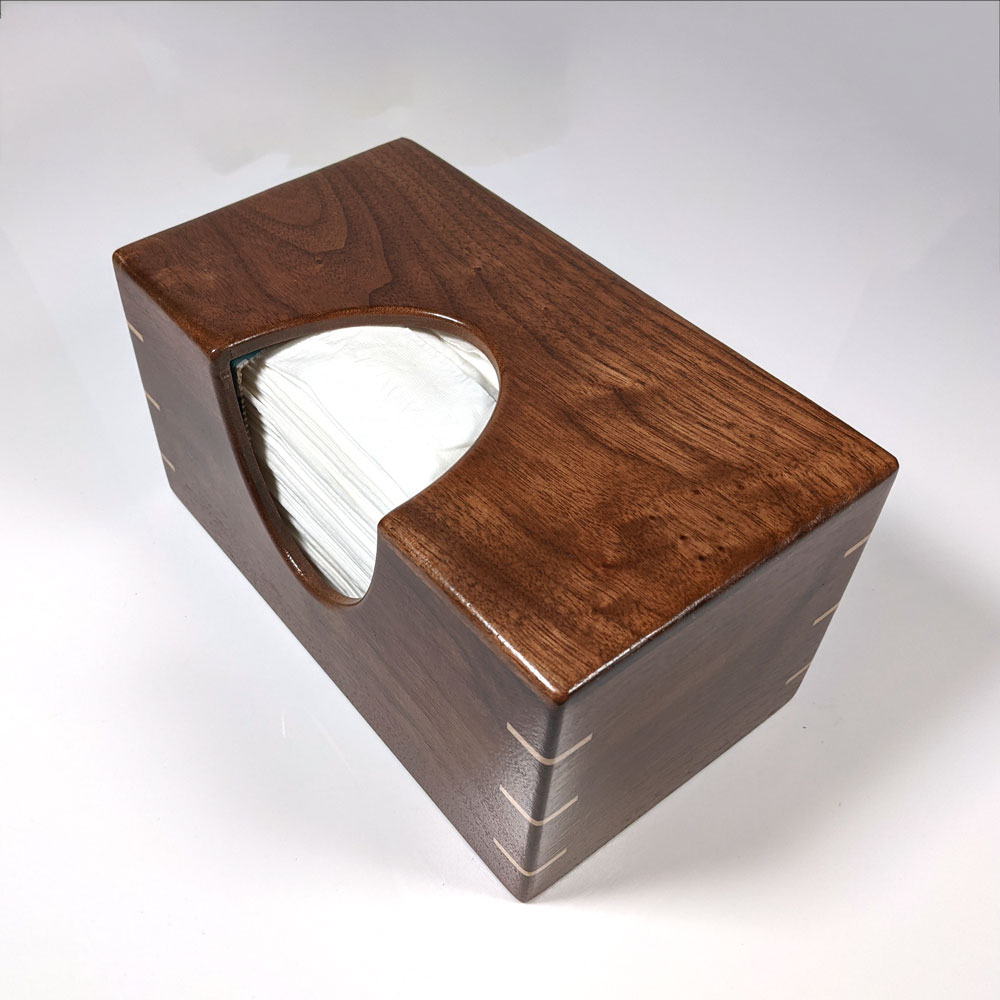This image features a custom-made tissue box crafted from elegantly dark-stained wood. The rich wood grains differ between the top and sides, with the top exhibiting a reddish hue and the sides displaying a warmer walnut color. Each of the box's three visible corners is adorned with symmetrical, decorative metal rivets, three per corner. Additionally, three lighter brown lines, resembling bands, accentuate each corner of the rectangular box. The tissue box is designed with half-circle openings on both the top and front for easy access to the white tissues inside, which lie flat, showing the contents through a perforated section on the left side. The edges of the box appear smooth and glossy, reflecting light. Positioned against a subtle gray gradient background, the box casts a faint shadow to the right, viewed slightly from above and over its front right corner. The overall craftsmanship highlights both functionality and aesthetic appeal, making it a distinguished decorative piece.